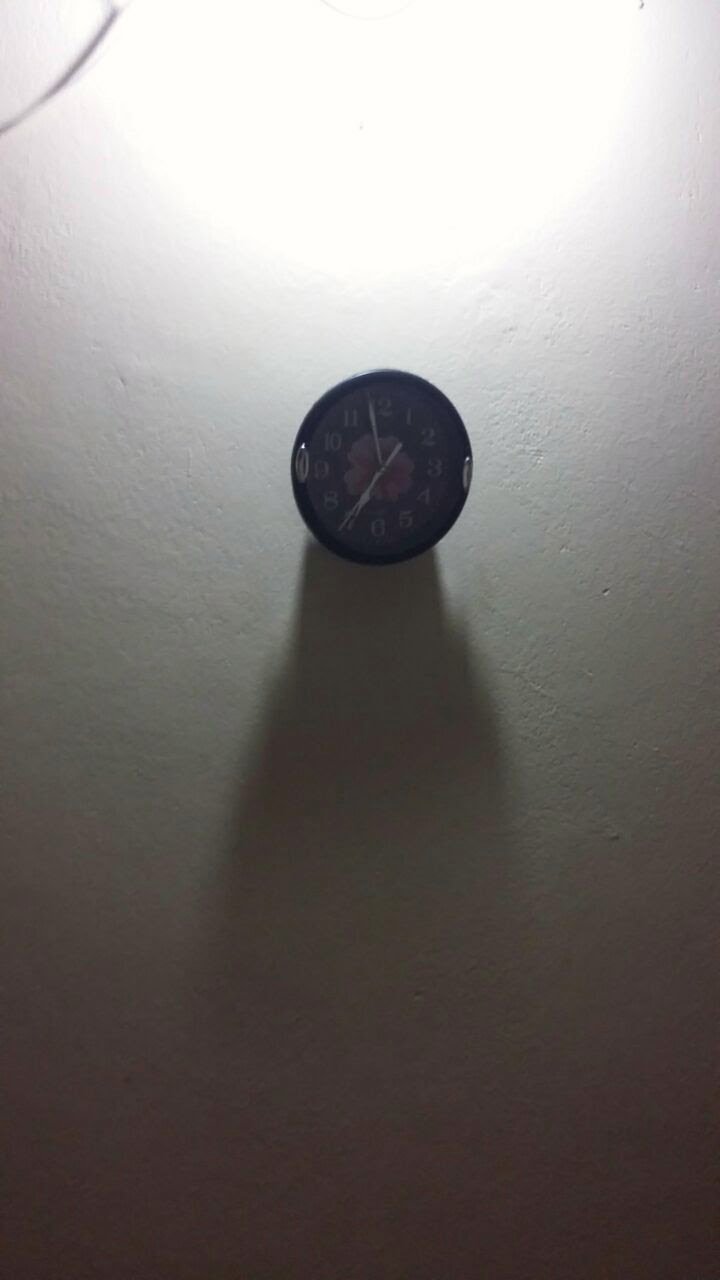This is a detailed color photograph of a small, round clock hanging on a slightly textured, white painted wall. The clock is prominently black, featuring white numerals from 1 to 12 around its outer rim and white hands, indicating the time as approximately 11:35. In the center of the clock face, there's a distinct image of a pinkish colored flower. A bright light source located at the top of the image casts a long shadow directly below the clock, adding depth to the scene. The overwhelming white background and the significant blank space below the clock gradually transition into a darker shadow area towards the bottom of the image, highlighting the minimalistic aesthetic of the photograph.